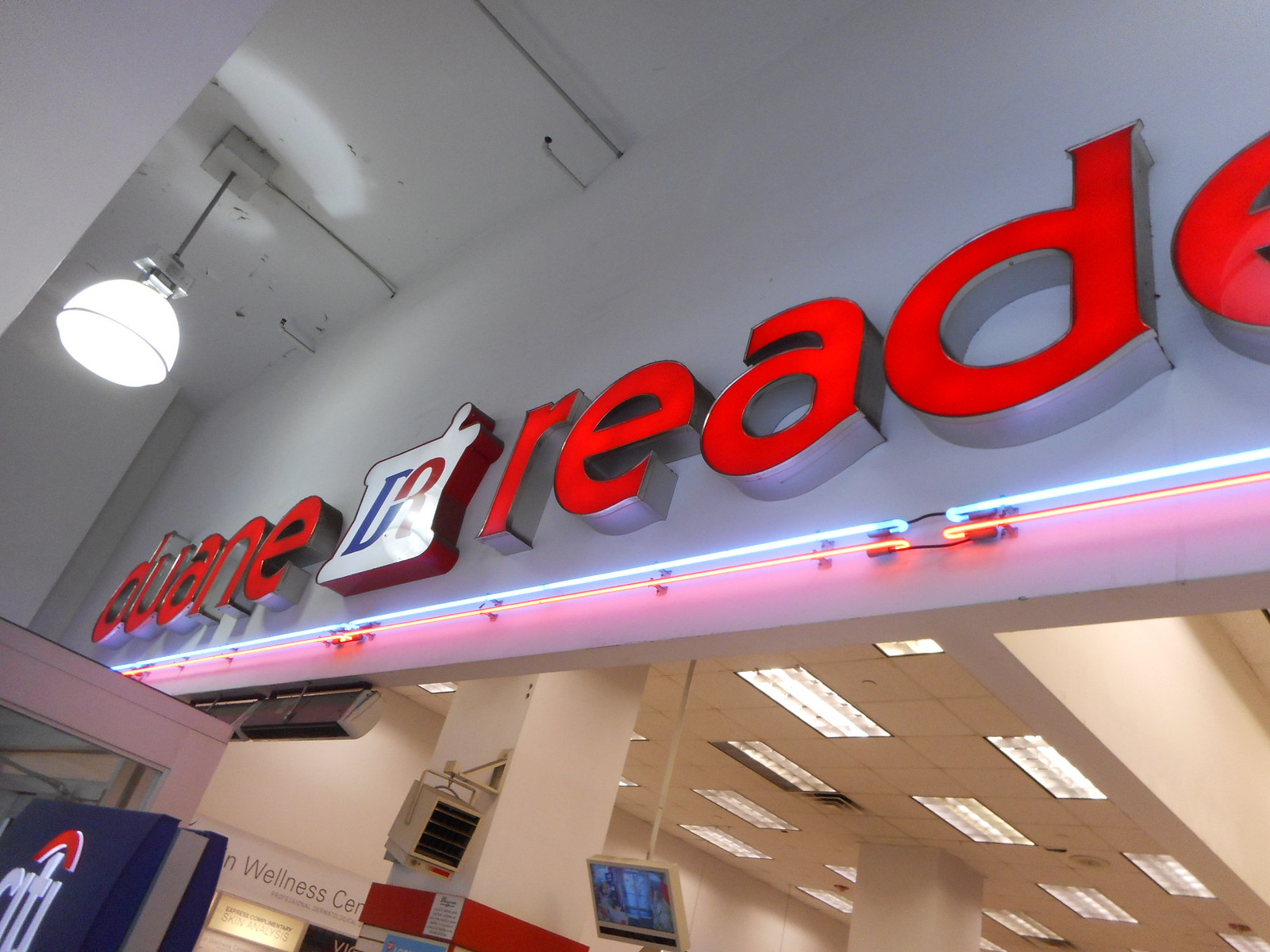The image captures the entrance of a Duane Reade pharmacy, prominently featuring the store's sign with the "DR" logo at the center. The logo is set against a white background, with a blue "D" and a red "R." Surrounding the sign are neon lights in blue and red, creating an inviting yet standard aesthetic for the pharmacy. Below the signage, there is a city ATM, emphasizing the convenience provided to shoppers. A sign labeled "Wellness Center" and a security camera hanging from the ceiling are also visible, ensuring both customer health and safety. The interior is brightly lit with fluorescent lighting, and the walls are predominantly white with accents of red paint. Various colored signage adds to the organized and welcoming atmosphere of the entrance. Overall, this is a typical pharmacy setup, offering a wide array of goods and services to patrons.